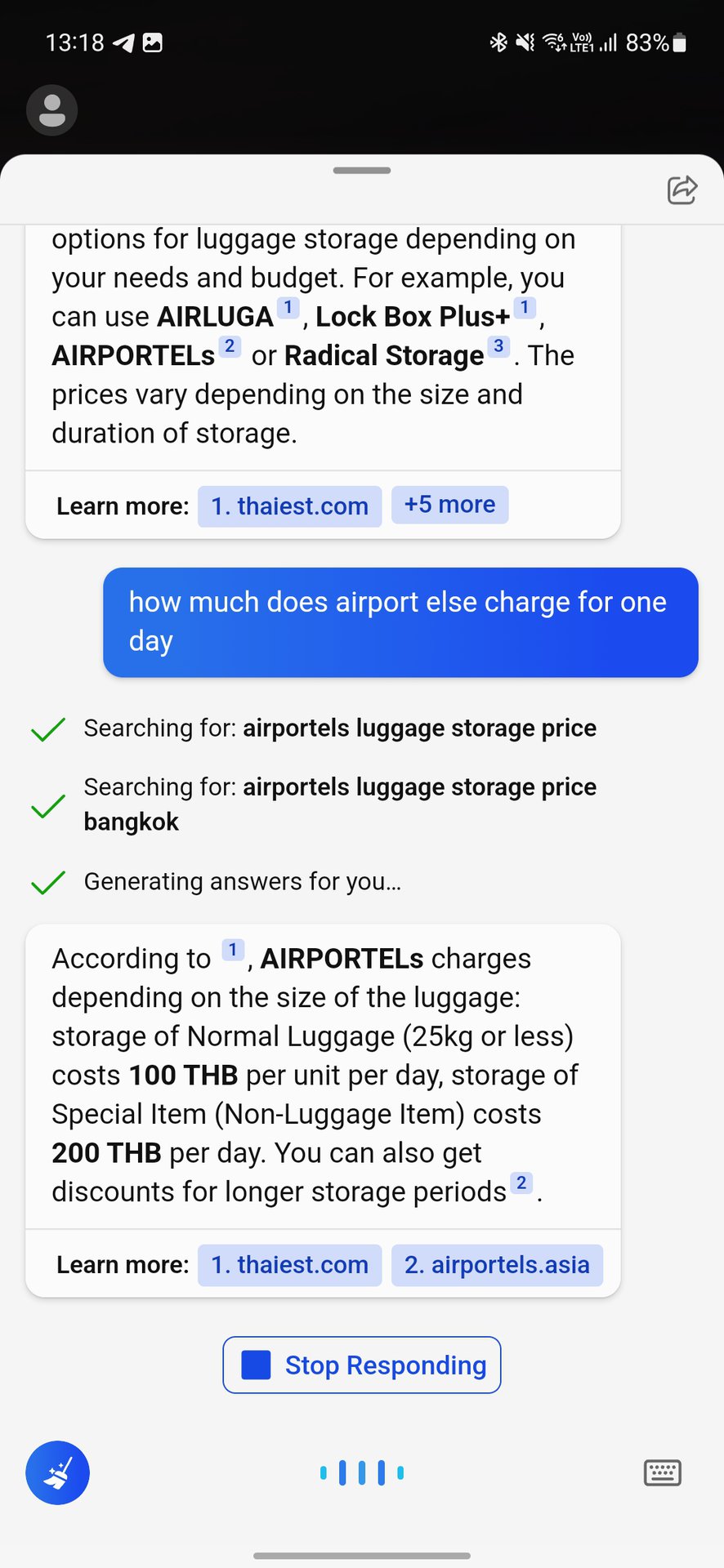The screenshot image showcases a list of options for luggage storage tailored to different needs and budgets. Featured services include AirLugga, Lockbox Plus, AirPortals, and Radical Storage, with prices varying based on the size and duration of storage required. Specific details regarding AirPortals are highlighted, with several green checkmarks indicating verified search results related to their pricing. For example, in Bangkok, AirPortals charges 100 THB per day for standard luggage weighing up to 25 kg, and 200 THB per day for special or non-luggage items. Additionally, discounts are available for extended storage periods. Further information can be found on bayeast.com and airportals.asia.